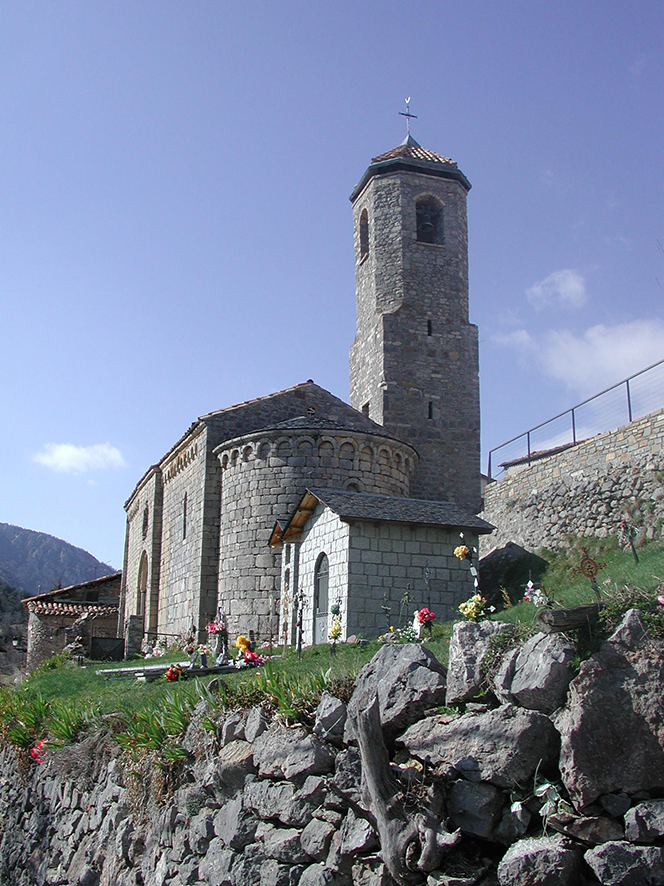The image depicts an old, majestic gray stone building that appears to be a church, characterized by its striking architectural features. Dominating the structure is a tall, pointed tower adorned with a wind vane and a cross at the top. Beside the main rectangular section of the building, there is a smaller, rounded section with a curved roof and an arched doorway, which adds to its castle-like appearance. In front, another more modest gray stone building with a slanted roof complements the scene.

The surrounding area is lush and green, with a well-maintained grassy patch and an array of multicolored flowers that seem to be carefully placed, suggesting it may be a cemetery where grave sites are decorated. Two stone walls frame the scene: one low retaining wall in the foreground and a taller wall with a railing behind the church, adding to the sense of enclosure and historical ambiance. In the background, the left side of the image features a glimpse of distant mountains beneath a clear blue sky with several wispy clouds. The entire setting is perched above a rocky slope, giving it an elevated, almost serene appearance.